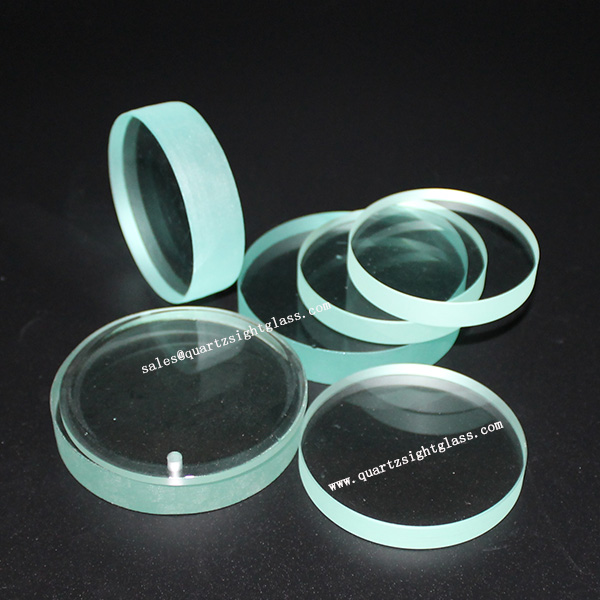The photograph features a striking display against a black, shiny background, showcasing six teal-colored glass discs. These discs, possibly lenses or lens covers with reflective glass centers, are arranged in various positions: three discs are stacked vertically, one stands upright on its edge, and two are lying flat. Two diagonal watermarks overlay the image: "sales@quartzsiteglass.com" in the center and "www.quartzsiteglass.com" closer to the bottom right, both inscribed in white text. The elegant teal rings and the meticulous arrangement emphasize a promotional or sales context for Quartzsite Glass products.